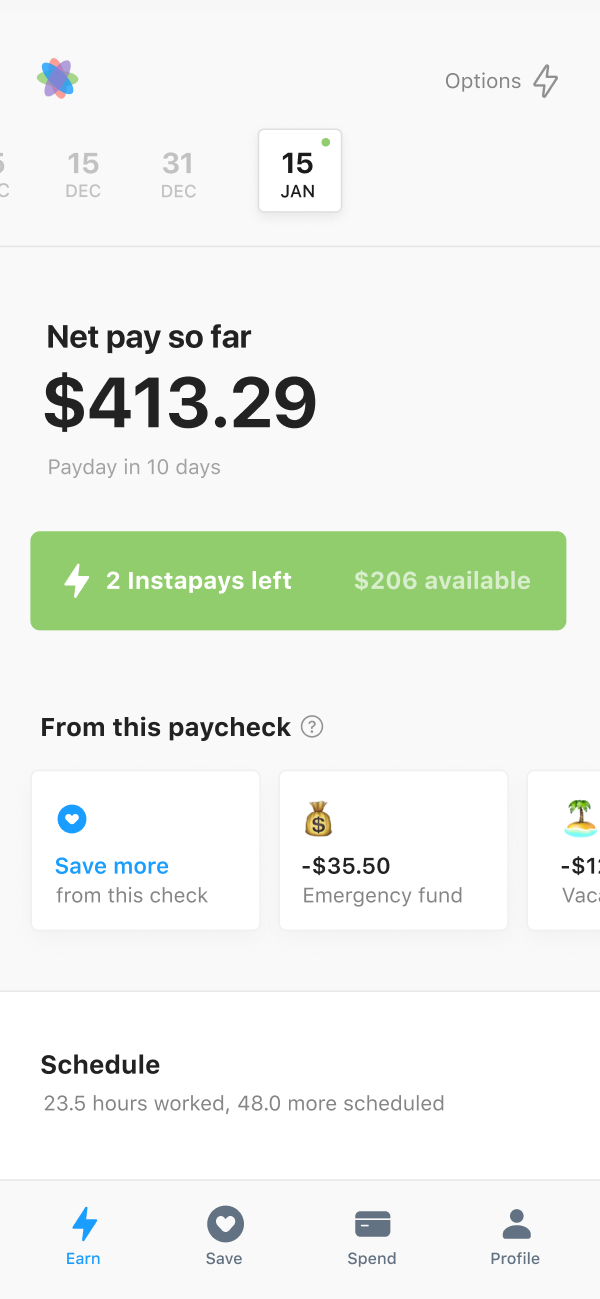The image is a screenshot from either a desktop web page or a mobile app interface displaying a payroll summary for an employee. The predominant background color is a muted grey. In the top section, several dates for pay periods are listed, specifically highlighting the pay period ending January 15th.

Centered prominently in bold black text is the statement "Net Pay So Far," followed by the amount "$413.29." Below this, in smaller grey text, it indicates "Pay Day in 10 Days," suggesting that the pay period has ended, but the pay day is still pending.

Beneath this information, there is a green rectangular box featuring a lightning bolt icon on the left side. The box contains white text reading, "2 Instapays left, $206 available," indicating the employee has access to two advance payments totaling $206.

Further down, the interface displays two smaller white boxes with corresponding icons: the left box encourages saving with the phrase "Save More from This Check," while the right box notes a deduction with the message "-$35.50 Emergency Fund."

Finally, towards the bottom of the screen, there's another rectangular box with the word "Schedule" in black text, which also notes in smaller grey text that the employee has worked 23.5 hours so far, with an additional 48.0 hours scheduled.

Overall, the image is a detailed snapshot of the employee's current payroll information, upcoming paycheck, and work schedule.